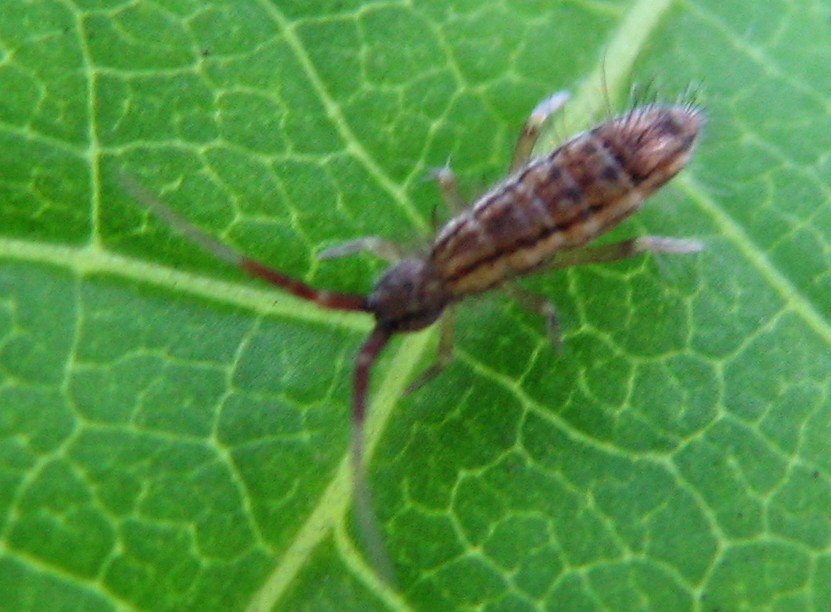A close-up, landscape-oriented photograph captures an insect perched on a bright green leaf. The surface of the leaf, which fills the entire frame, is detailed with prominent veins that run from the top right to the bottom left, accompanied by smaller branching veins in light yellow. The insect, centrally positioned but slightly facing down and to the left, appears to be a beetle. Its body is elongated and oval-shaped, shaded in various tones of brown with darker spots in the middle, and features a tuft of hair at the rear. Its head is small, round, and slightly grayish-brown, equipped with six nearly translucent gray legs bent at the knees. The most striking features are the insect’s long antennae, spreading out divergently at approximately 45-degree angles; they are dark brown near the head and fade to a lighter gray toward the tips. Despite the overall blurriness of the image, the detailed structure and colors of the insect and leaf are discernible, emphasizing the photographic realism of the scene.